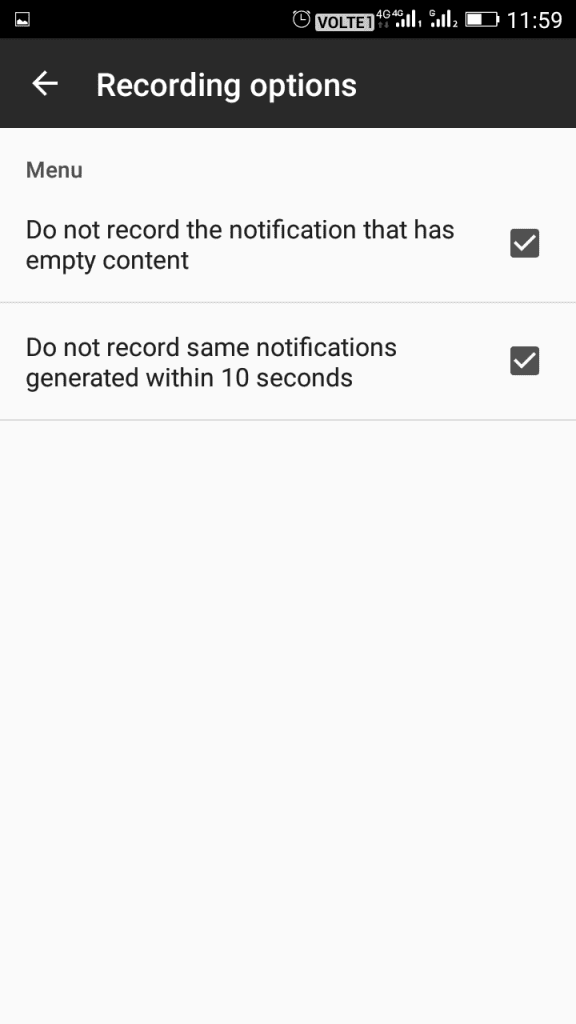A detailed screenshot taken from a smartphone displays various interface elements. At the very top, a black banner houses several icons. On the far left is a small white square icon resembling a home or mountaintop, with an unclear purpose. Centrally aligned from the left is an alarm clock icon and "Volt T1," followed by a 4G signal indicator, a G signal icon, and a battery icon showing approximately 50% charge. The time on the far right reads 11:59.

Beneath the black banner, a wider, grayish-shaded panel contains white text related to recording options. Below this panel, on the left, a heading in gray reads "Menu." In a slightly larger font, the text specifies, "Do not record the notification," with an empty content section beneath it. To the right of this text is a ticked checkbox. A fine gray line separates this section from another option below, which reads, "Do not record same notifications generated within 10 seconds." This option also has a ticked checkbox beside it.

The image concludes with another fine gray line beneath the second option, leaving the rest of the screen as a plain white background. (Note: A promotional line for Beadaholique.com seems to be inadvertently included in the caption but has no relevance to the screenshot details).